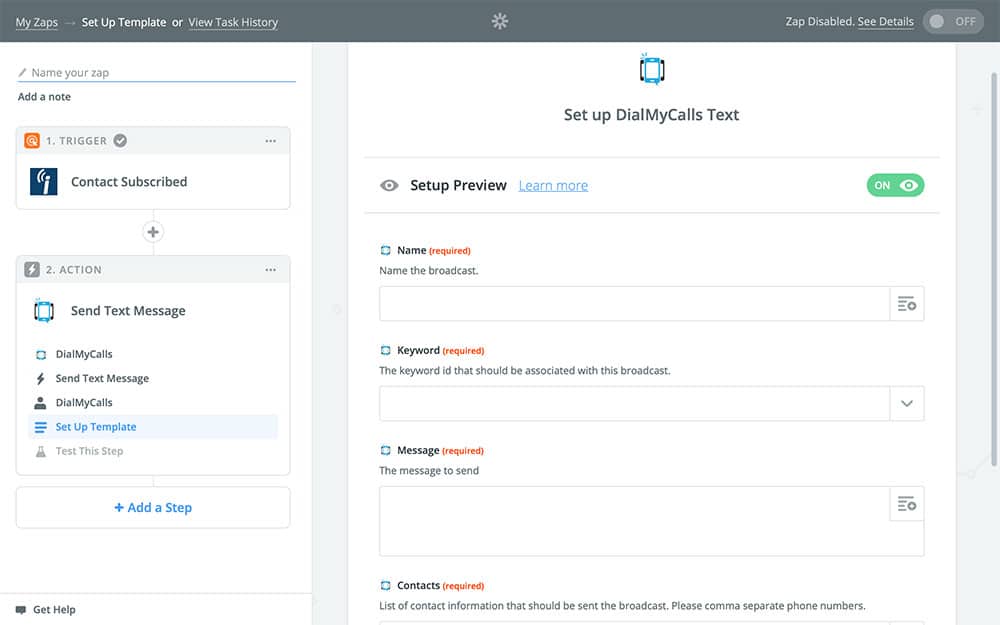**Detailed Caption:**

The image depicts a web page interface for a service called "Zap." At the very top, there's a gray navigation bar. From left to right, this bar includes the options "My Zaps," followed by "Set Up Template" and "View Task History," which are spaced evenly apart. These options appear in a grayish-white font. In the center of the bar, there is a small gray flower icon. On the right side, the bar displays the text "Zap Disabled," which is underlined and followed by "See Details." Additionally, there's a switch that appears to toggle something on and off. 

Below this gray bar, on the left, there is a section labeled "Name Your Zap" in gray text. Next to it is a blue line, followed by an option to "Add a Note." 

In the main section of the page, a box features an icon and the text "1. Trigger," highlighted by a checkmark and three dots for more options. Beneath this, in a white background, there's a blue icon next to the text "Contact Subscribed."

Further down, a small plus sign adds another section. Below this, another gray bar houses an energy icon and the text "2. Action." This section details "Text Send Text Messages," with smaller text below reading "Dial My Calls." Options include "Send Text Message," "Dial My Calls Again," "Set Up Template," and "Test This Step."

At the bottom of this box, there's a blue link that says "Add a Step." On the right side, the text reads "Set Up My Text with Dial My Calls." Above this text, there's a small icon and the headings "Set Up," "Preview," and in blue, "Learn More." Here, there’s another toggle switch.

Further down the page, fields for "Name" (required), "Keyword" (required), and "Message" (required) are provided to name the broadcast, specify a keyword ID, and compose the message to be sent, respectively. At the very bottom, there's an instruction section for "Contacts" (required), detailing to list contact information for the broadcast, with directions to comma-separate phone numbers. This section extends beyond the viewable area of the image.

This comprehensive layout provides a clear workflow for creating and managing Zaps, complete with triggers, actions, message settings, and contact information.